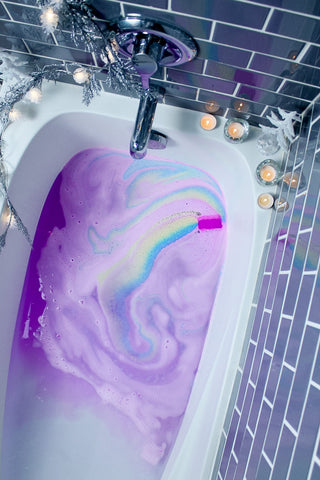The image showcases a relaxing and artistic bathtub scene, captured from a bird's-eye view. The bathtub, which is white and occupies the central focus of the image, is partially filled with water displaying a mesmerizing swirl of colors. Predominantly, the water is a gradient of lavender to dark purple, with striking streaks of yellow, blue, and hints of green, reminiscent of a vibrant rainbow within a purple cloud. Surrounding the tub, the black subway tiles with white grout provide a sharp contrast, enhancing the visual appeal of the scene.

Accentuating the soothing atmosphere, several lit candles are strategically placed around the edges of the bathtub, emanating a warm, inviting glow. The chrome-finished faucet and silver overflow valve add a touch of elegance, while a green sprig adorned with white balls lends a natural, spa-like feel to the setup. This serene and well-composed image captures the essence of a luxurious and tranquil bathing experience.